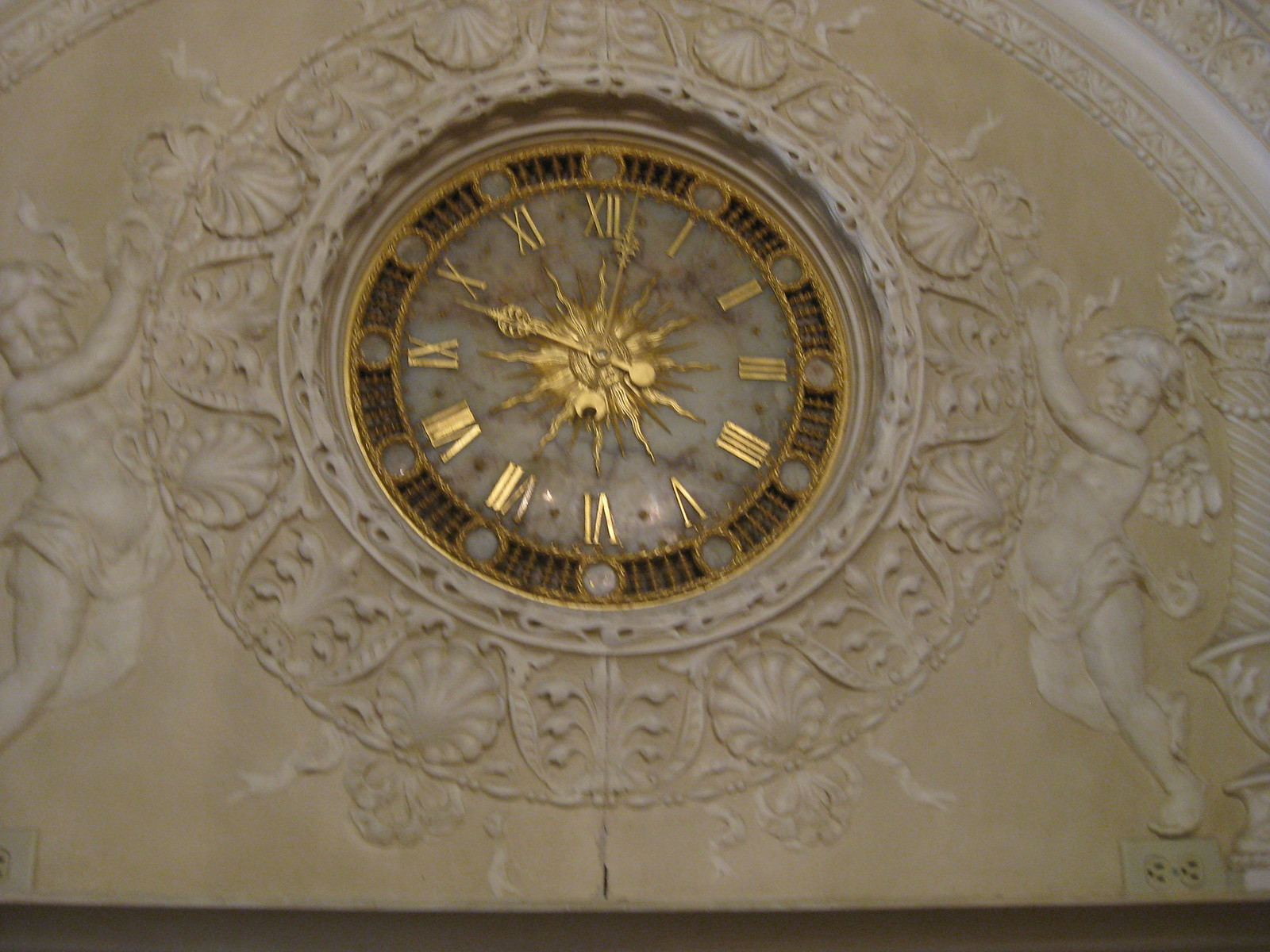The image depicts a grand and ornate clock set into a smooth stone wall, likely part of a clock tower, church, or a grand museum. The clock features a circular golden frame with Roman numerals and is set against a backdrop of intricate shell carvings. At the heart of the clock is a fiery gold sun motif from which the gold hour and minute hands extend. The stone surrounding the clock is clean and smooth, forming an archway shape. Flanking the clock on either side are two cherubic figures or infants facing each other, contributing to the overall decorative and historical feel of the piece. Notably, in the bottom right corner of the frame, beneath one of the cherub’s feet, there is a modern electrical outlet, suggesting the clock's installation on an interior wall. The photograph has a yellowish tone and is somewhat grainy, indicating either the age of the photo or the use of a filter. The time displayed on the clock appears to be around 10:10.